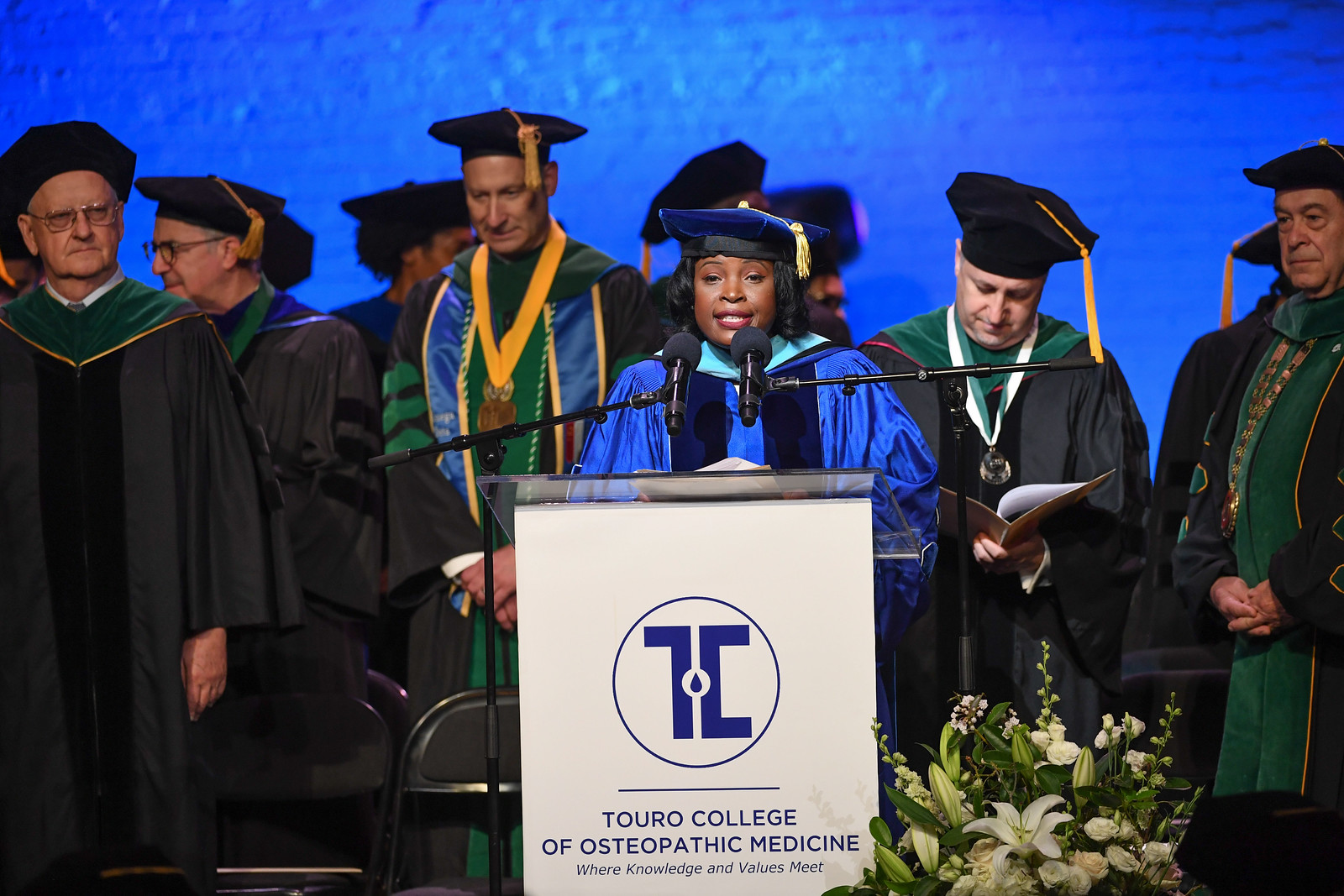In this detailed image, a black woman with short dark hair stands behind a podium on a stage, dressed in a blue graduation cap and gown, complemented by a darker blue ribbon draped around her neck. The podium front features the logo of Touro College—a T and a C encapsulated in a circle, resembling an upside-down L with a teardrop—and bears the inscription "Touro College of Osteopathic Medicine: Where Knowledge and Values Meet" in blue text on a white background. Positioned prominently, two microphones are directed towards her, suggesting she might be speaking or presenting.

Behind the woman, several rows of individuals sit, presumably professors or graduates, all donned in black gowns with green V-shaped collars featuring yellow trims. Their black graduation caps uniformly sport tassels pointing to the left. In the first row and visible parts of the second and third rows, most of the seated men can be seen, with one man to the left of the main speaker wearing a yellow ribbon around his neck attached to a medal. Another individual on the right side of the image also sports a medal around his neck. At the bottom left of the photo, there are empty black chairs, and to the bottom right, adjacent to the podium, a bouquet of white flowers with green leaves adds an elegant touch to the scene.